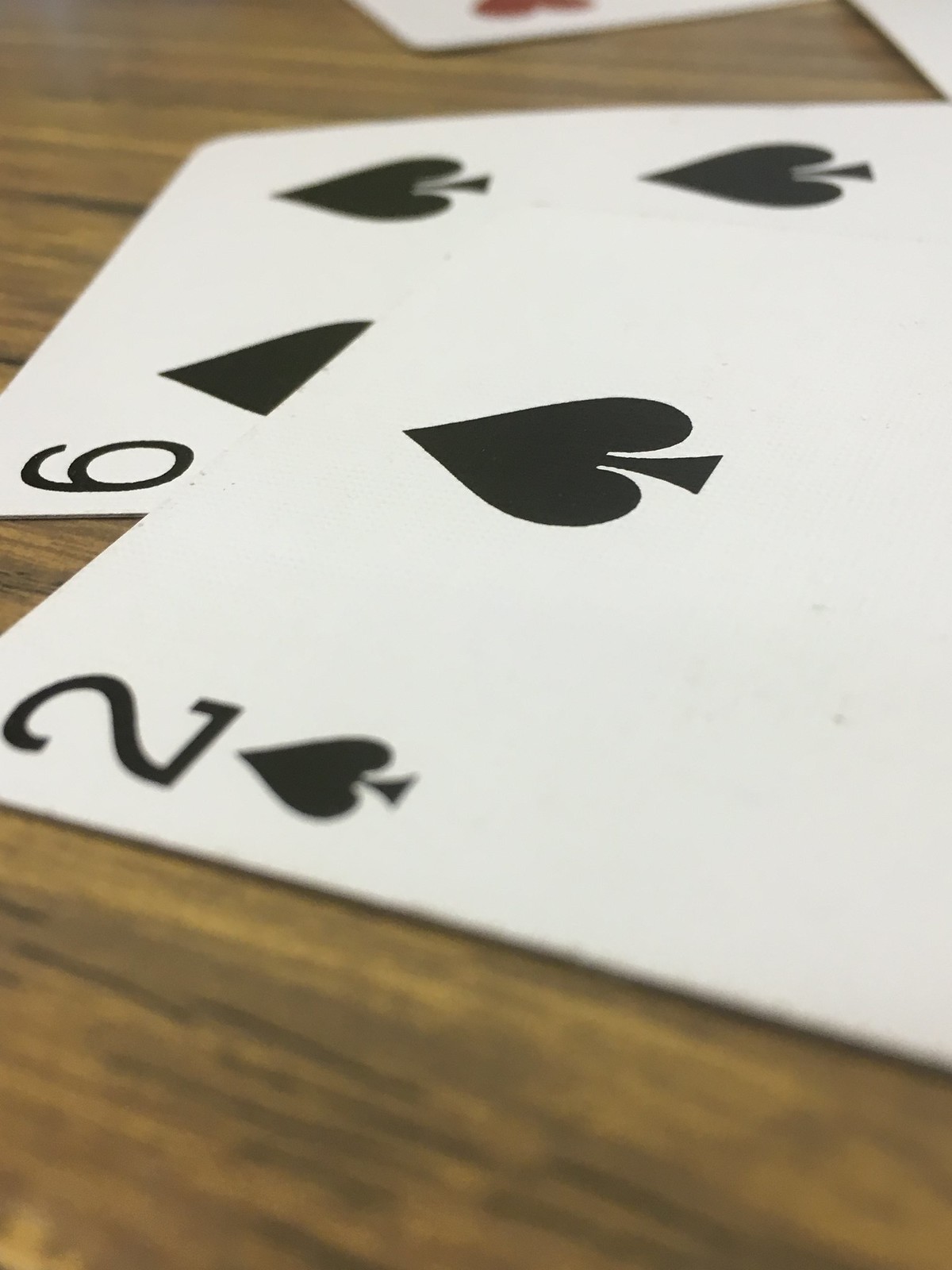This captivating macro photograph, taken in portrait mode, offers an intimate close-up of two playing cards against a richly textured wooden background. The wooden surface exhibits a dynamic range of dark, nearly black-brown to light yellowish hues, providing a warm, natural context. Dominating the foreground is the two of spades, its recognizable black spade symbol slightly out of focus, adding depth to the composition. Directly beneath it, the six of spades stands in sharp focus, showcasing its crisp, black markings against the plain white card. In the distant background, a hint of a red card peeks into the frame, its identity obscured by an intentional blur. Additionally, a barely discernible edge of another card appears at the top right corner, further contributing to the enigmatic ambiance of the photograph. This image skillfully balances clarity and mystery, capturing the viewer's attention through its meticulous focus and rich, natural textures.